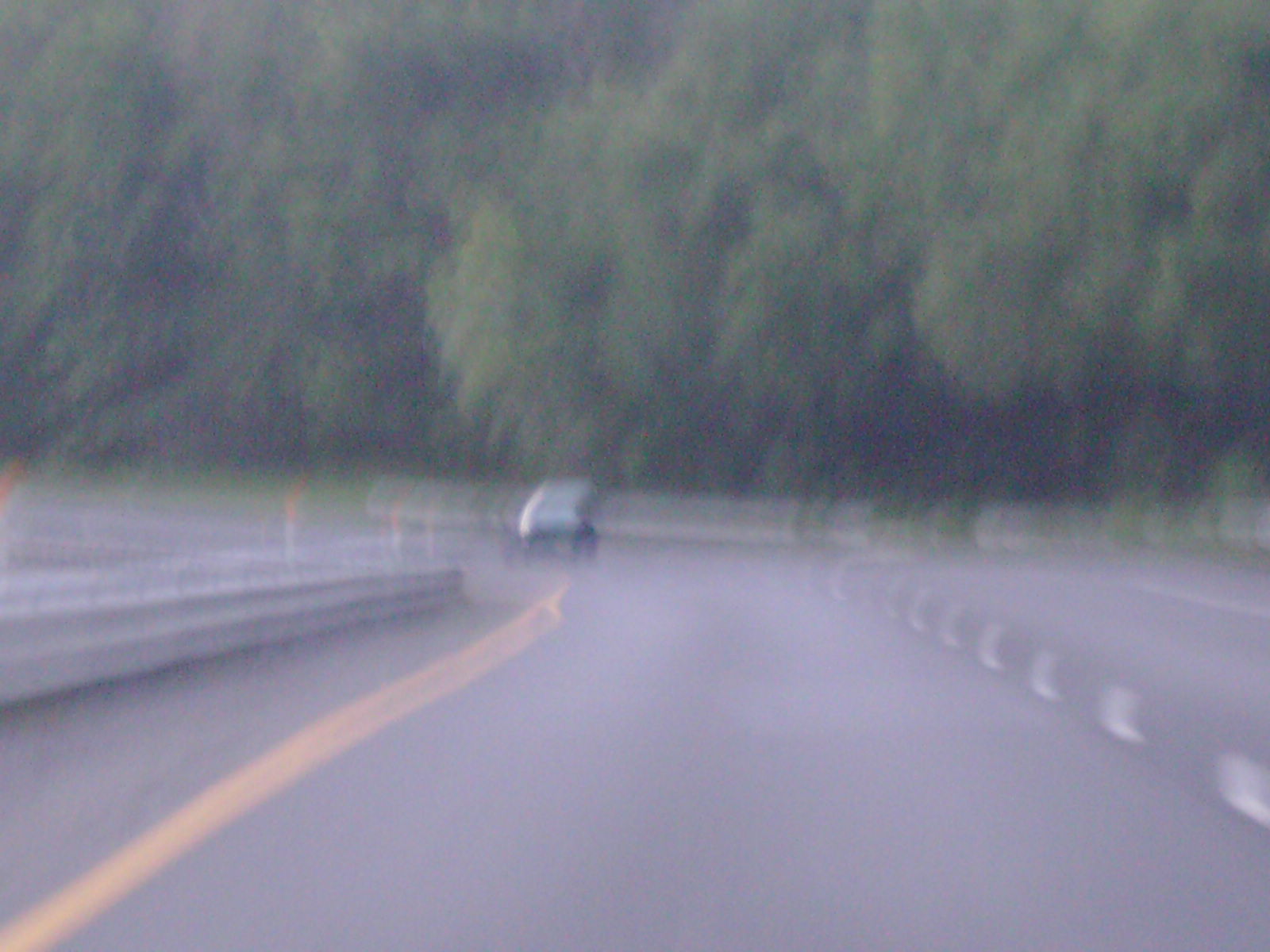The photo presents a dynamic scene of a highway journey, viewed from the perspective of a vehicle moving along the road. The entire image is characterized by a motion blur, which gives it an impressionistic quality. The highway itself is an asphalt road that occupies the lower half of the image up to its midpoint. The road features two lanes, and the vehicle from which the picture is taken is traveling in the left-hand lane. Ahead, the road curves sharply to the left mid-frame.

A dark-colored car is visible in front of the observer's vehicle, although its make and model remain indeterminate due to the blur. The curvature of the road towards the left is accompanied by a lush, verdant bank of trees that fills the upper portion of the image. These trees display a mix of light and dark green foliage, adding a dense, natural backdrop to the scene.

To the left of the image, there is an indistinct structure that could possibly be a central reservation or a divider. The exact nature of this divider is ambiguous due to the image's overall blurriness. This ambiguity also introduces a question about the highway's geographical location and traffic orientation. It raises the possibility that the image might depict a dual carriageway, with the observed vehicle traveling on the right side of a divided highway, suggesting a country where driving on the right is customary.

In summary, the photo captures a blurred yet detailed scene of a highway journey, with a sharp left curve, a leading dark vehicle, and a dense background of foliage. The indistinct central structure adds an element of mystery regarding the road's layout and the geographical driving norms.